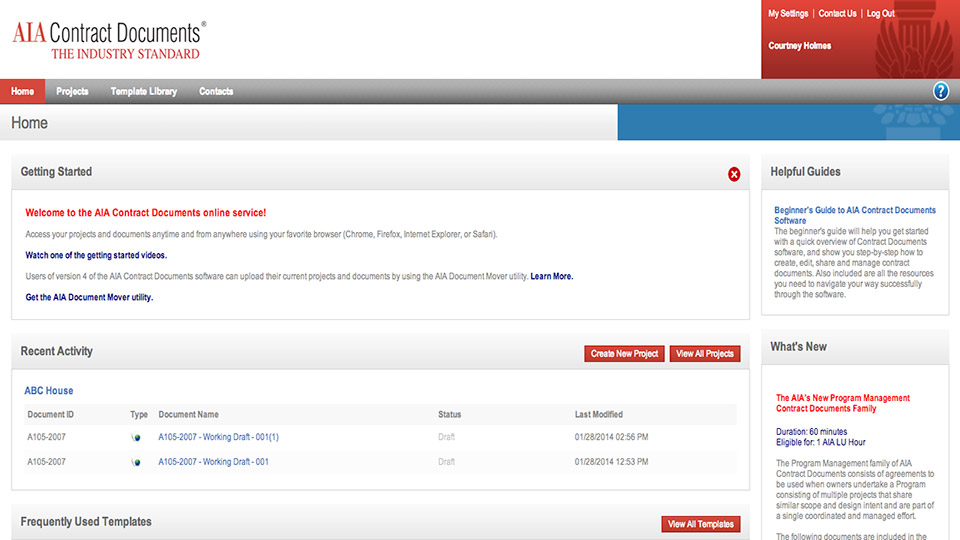The screenshot captures the homepage of the AIA Contracts website. On the left side of the page, just underneath the "Contract Documents" header, the text "The Industry Standard" is prominently displayed within a red triangle. To the right of this, user-specific options including "My Settings," "Contact Us," and "Logout" are visible next to the user's name, Courtney Holmes.

Directly below, a navigation bar or dock displays menu options such as "Home," "Projects," "Template Library," and "Contracts." The "Home" tab is highlighted in red, indicating it is currently selected, while the others remain in gray.

Continuing down, a secondary navigation bar includes the "Home" tab, mirroring the top navigation and complemented by a blue end bar. At the very top of the content area, there is an introductory section labeled "Getting Started," which can be dismissed with an 'X' icon. This section welcomes users to the Documents Online Service, providing links to instructional videos to aid beginners, suggesting that some training might be necessary.

Below this introductory section, the "Recent Activity" section lists options to "Create New Project" or "View All Projects." Under this, there is a display of recent documents with titles such as "ABC House" and other document names, followed by a section named "Frequently Used Templates" and an option to "View All Templates."

Additionally, the homepage features two informative articles: "Beginner's Guide to AIA Contract Document Software" and "The AIA's New Program Management Contract Documents."